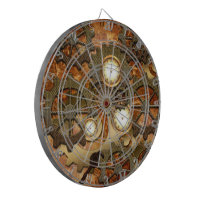The photograph features a piece of wall art, styled like a steampunk-inspired dartboard, set against a clean, white background often used for commercial purposes such as online shops or catalogs. The circular art piece, seemingly floating due to the edited out background, is angled slightly to the right, revealing both its front and sides. It’s encircled by gray edges and features multiple concentric rings, with a small rope or metal hook at the top, forming an inverted V for hanging.

At the center of the dartboard-like design, three white-faced clocks with gold rims are arranged in a triangular pattern; one clock is positioned at the top, while the other two sit lower and to the sides. The art is rich in detail, displaying a pattern of creams, greens, oranges, reds, and browns, alongside intricate lines and cogs that evoke a sense of mechanical complexity. The outermost ring is marked with numbers, likely intended to mimic the scoring system of a traditional dartboard. This detailed, multi-layered piece seamlessly blends aesthetics with function, making it a distinctive artifact that captures the essence of steampunk design.